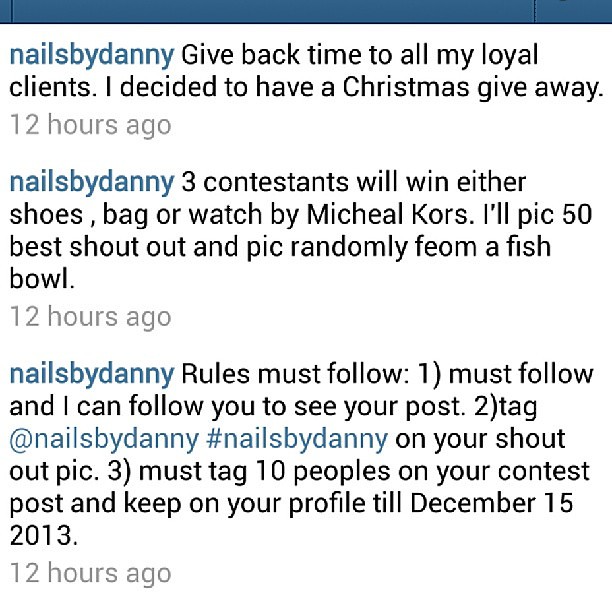This is a screenshot likely from an Instagram post by Nails by Danny. At the very top, a blue rectangular line is visible. The text on the white background is a mix of black, blue, and gray. The post, made 12 hours ago, details a Christmas giveaway for loyal clients. Three contestants have the chance to win a pair of shoes, a bag, or a watch by Michael Kors. Danny will choose the top 50 shout-outs and draw winners randomly from a fishbowl. The rules are outlined: (1) follow Nails by Danny to be followed back and have your post seen, (2) tag @NailsByDanny and use the hashtag #NailsByDanny in your shout-out picture, (3) tag 10 people in your contest post and keep it on your profile until December 15, 2013.